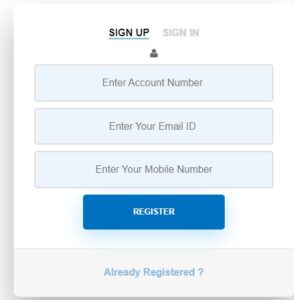The screenshot shows a pop-up window from a website. The pop-up appears against a light gray, slightly thicker background, positioned either on the left or right side. The main section of the pop-up is a white square with "SIGN UP" in bold, black capital letters at the top, underlined with a blue-gray line. Below "SIGN UP," in a subtle faded gray, is the text "Sign in." 

Underneath the text headers, there is a dark gray graphic depicting a head and shoulders icon. Below this icon, there are three blue banners, each containing a distinct option for user input: "Enter account number," "Enter your email ID," and "Enter your mobile number."

At the bottom of the pop-up, there is a bright medium to dark blue rectangle with the word "Register" in white text. The very bottom of the pop-up features a light gray background with light blue text that reads "Already registered?" followed by a question mark.